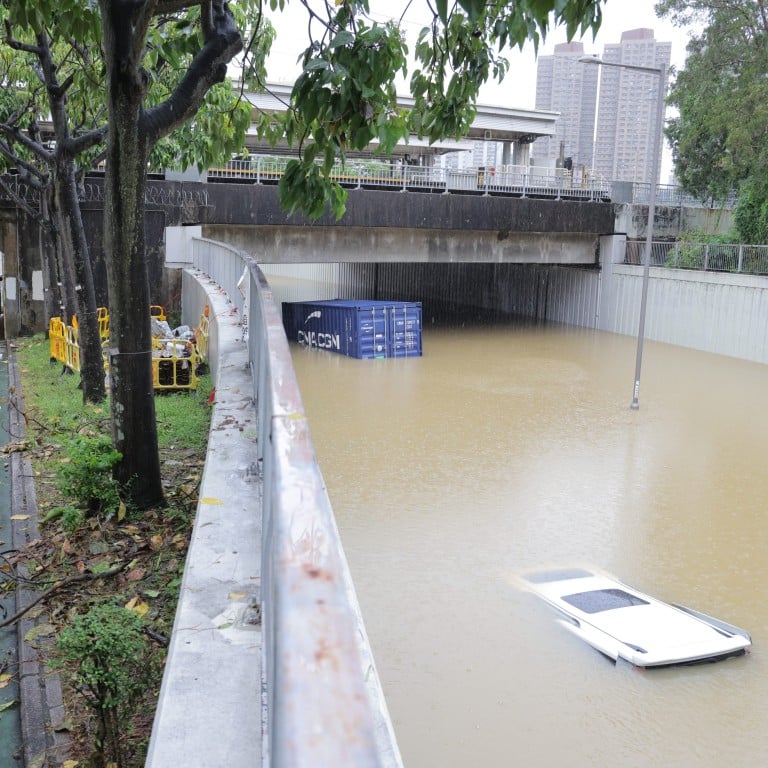This daytime city scene captures a severely flooded road that appears to run under a concrete bridge with a distinctive white railing on top. The floodwaters engulf a large box truck halfway up its container, while a white SUV is almost completely submerged, with only its roof and sunroofs visible above the water's surface. To the left side of the image, there are trees, grass, and what seems to be construction gates surrounding a collection of supplies. In the background, two tall buildings, possibly apartment skyscrapers or business towers with numerous windows, stand prominently. The image suggests that the road, resembling a canal or drainage area, has experienced significant flooding.